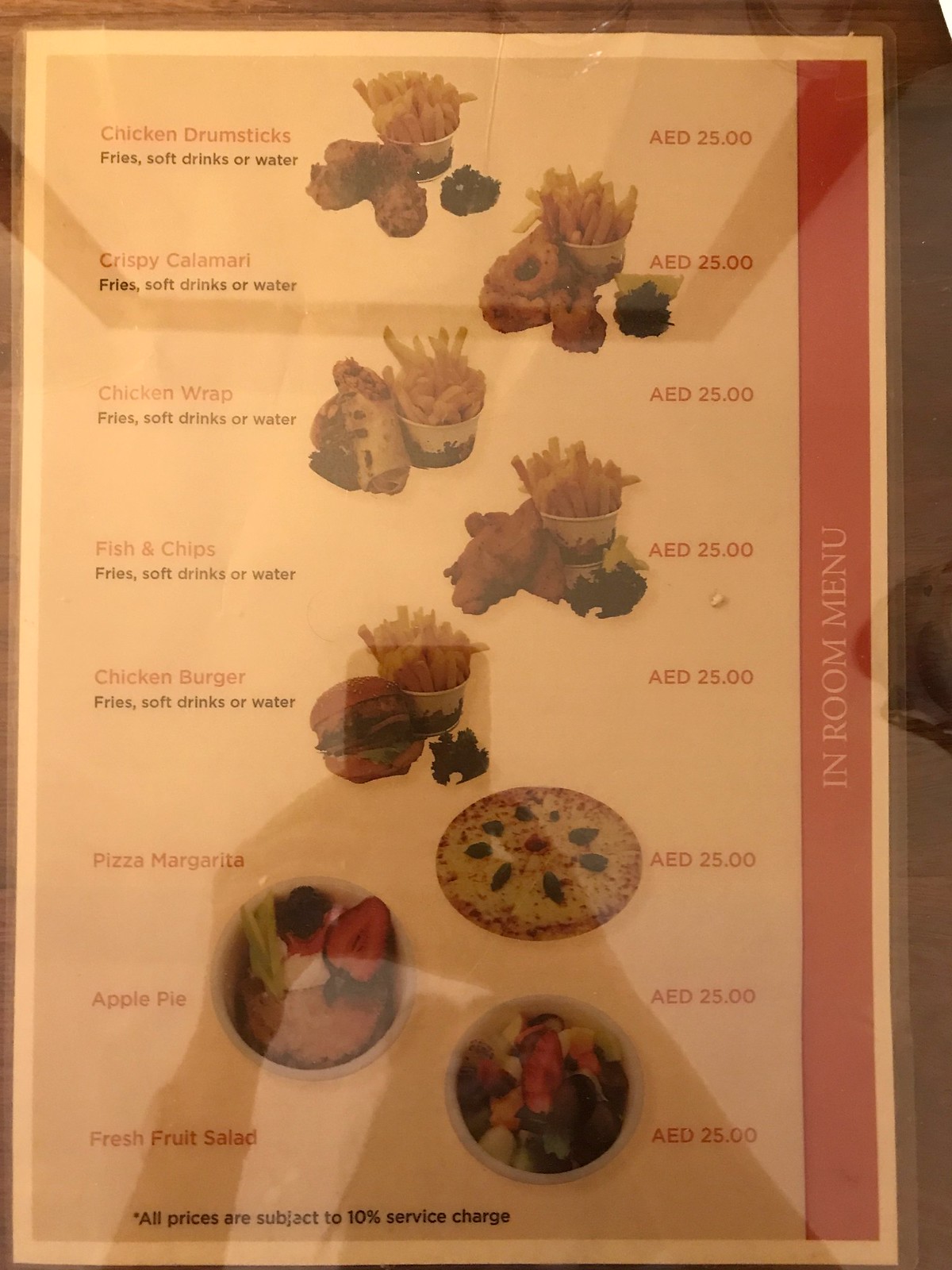This dimly lit photograph showcases a hotel room service menu encased beneath a translucent layer of lamination. The illumination is so poor that what would normally appear as a white menu has taken on a light orange hue. The menu is adhered to an unidentified surface, possibly a wall or a tabletop within the room, but the indistinct background makes it unclear.

The menu features a variety of items available for guests to order, each accompanied by a small graphic depiction of the corresponding dish. Starting from the top left corner, the listed items include:
- Chicken drumsticks with fries and a choice of either a soft drink or water, depicted with an image.
- Crispy calamari with fries and a choice of either a soft drink or water, also with an image.
- Chicken wrap with fries and a choice of either a soft drink or water, shown with an image.
- Fish and chips with fries and a choice of either a soft drink or water, illustrated with an image.
- Chicken burger with fries and a choice of either a soft drink or water, accompanied by a picture.
- Pizza Margherita, represented with an image.
- Apple pie, depicted with an image.
- Fresh fruit salad, shown with an image.

Despite the unclear setting and dim lighting, the menu’s detailed illustrations and variety of meal options are evident.